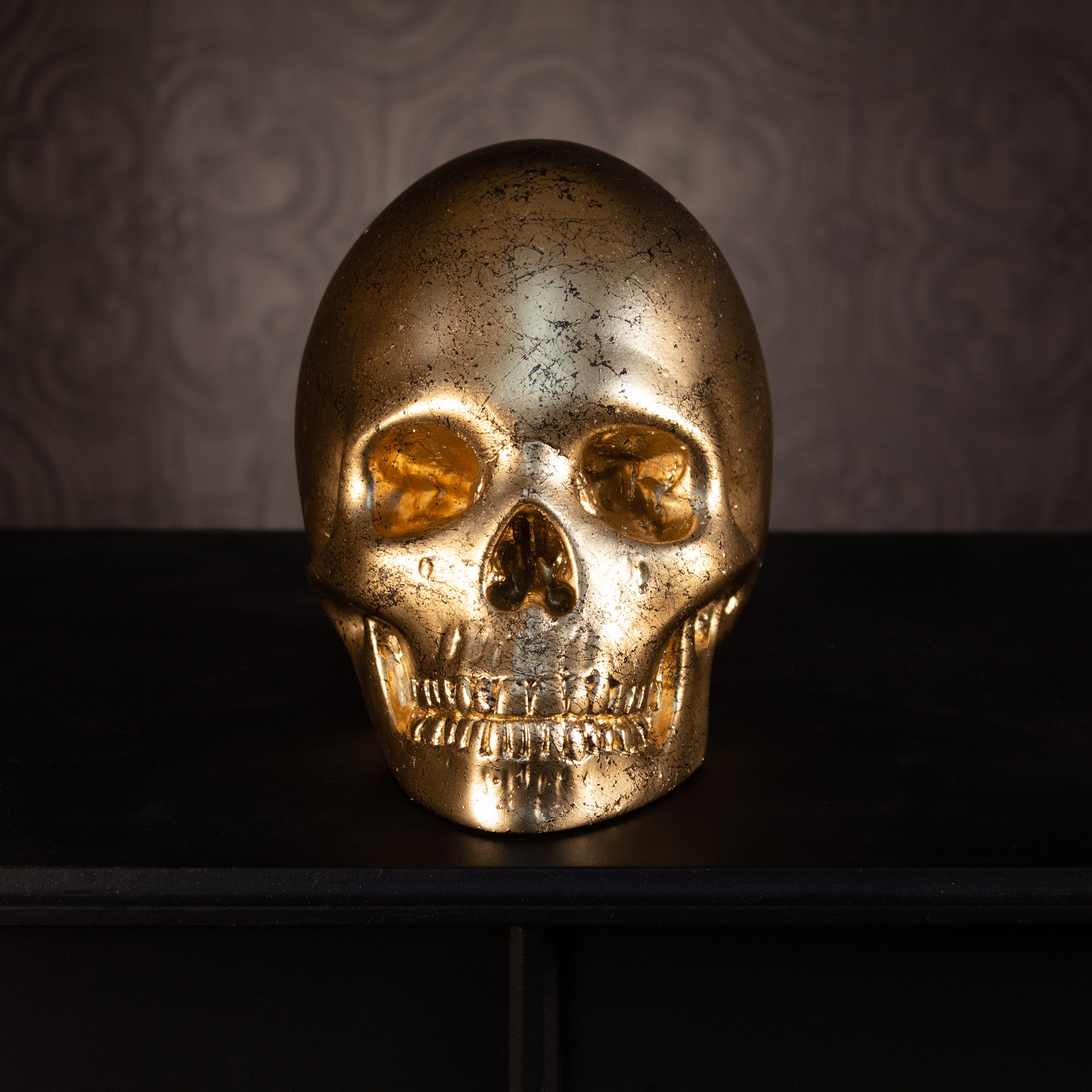This detailed color photograph showcases an intricately crafted metallic human skull, likely made of brass or a gold-toned plated material, exhibiting a weathered and aged look. The surface is brilliantly reflective, casting subtle light from the surrounding environment, with areas of black tarnish enhancing its antique effect. The eye sockets are notably polished, offering a stark contrast to the dark, empty nasal cavity. The teeth and jaw are stylized and fused together, presenting a cohesive sculptural form rather than individual elements. The skull is positioned on a dark surface, likely a black or dark brown chest of drawers, with an elegant mauve-brown floral patterned wallpaper in the background, adding an ornate and vintage aesthetic to the scene.